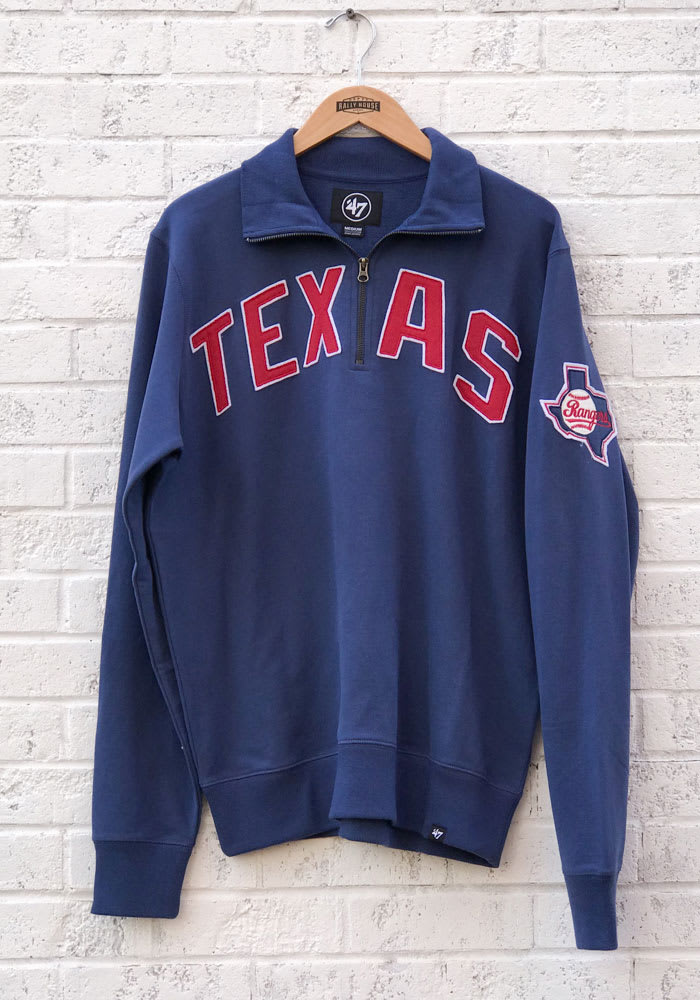The image showcases a navy blue, long-sleeve, zip-up Texas Rangers sweatshirt hanging on a wooden hanger, which is attached to a nail on a white-painted brick wall. The sweatshirt features red text across the chest with "TEX" on the left side of the zipper and "AS" on the right, spelling out "Texas." The right sleeve displays a white outline of the state of Texas with a red inner outline and a white baseball with red stitching, over which "Rangers" is written in red. The hanger appears to have a silver hook leading into a wooden body, possibly labeled "Rally Horse." Additionally, the black tag inside the collar showcases the number "47" in white within a circle. The image resembles a product photo, likely highlighting the sweatshirt's features and design details.